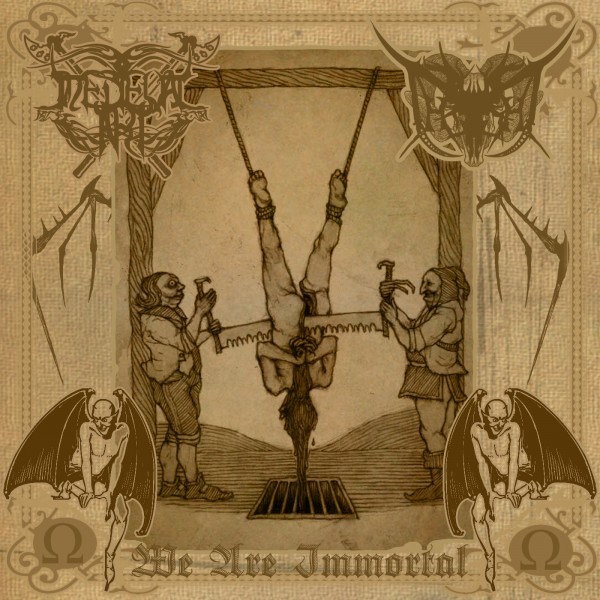This intricate sepia-toned medieval-style drawing is a graphic and disturbing depiction of a man being sawed in half while hanging upside down from a wooden structure. Bound by ropes tied to his ankles, the man is suspended over a grate into which his blood is flowing as two men, one on each side, grimly maneuver a two-man saw through his body from the groin downwards. The composition is further adorned with macabre details, including devilish or gargoyle-like figures with bat wings placed in the bottom left and right corners. Elaborate decorations frame the horrifying scene, which is underscored by an ominous inscription at the bottom: "We are immortal."